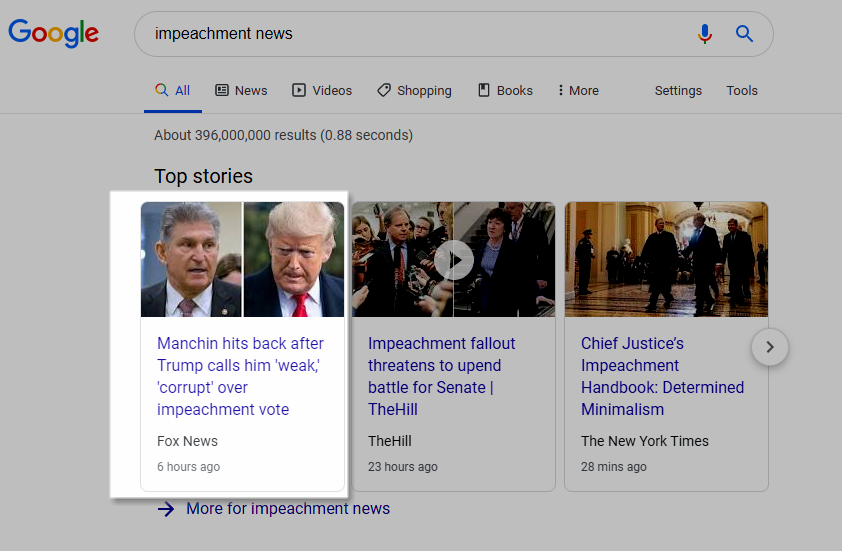The image captures a Google search results page specifically filtering news related to "impeachment". Dominating the screen are three highlighted stories. The lead article, prominently featured in white, is from Fox News, titled "Manchin hits back after Trump calls him 'weak,' 'corrupt' over impeachment vote," published six hours ago. Adjacent to this, The Hill presents a headline reading "Impeachment fallout threatens to upend battle for Senate," timestamped 23 hours ago. On the far right, the New York Times contributes with "Chief Justice's impeachment handbook determined minimalism," mere 28 minutes old. An arrow icon beside the New York Times article indicates there are additional stories available beyond these primary results.